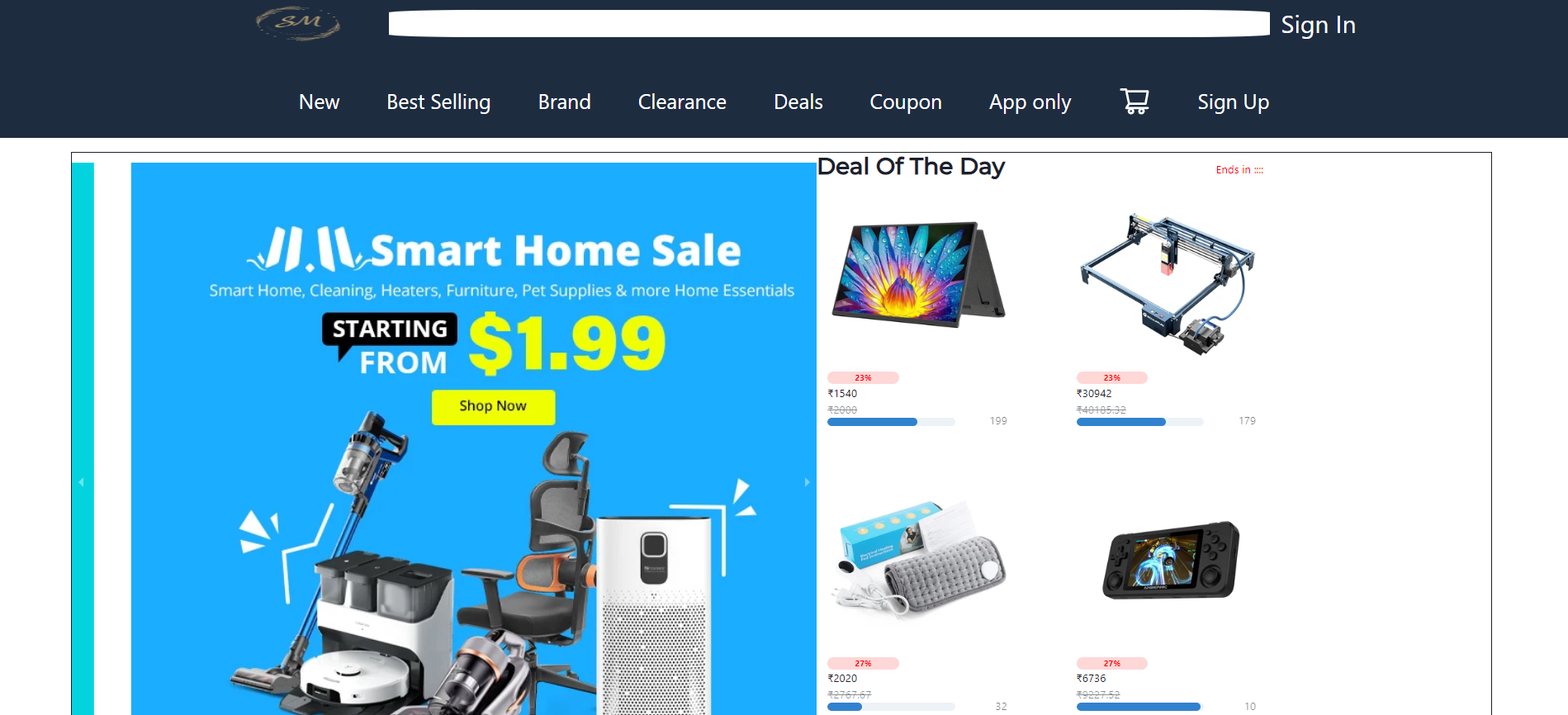**Detailed Caption for Desktop Screenshot:**

The image is a screenshot of a web app showcasing what appears to be an e-commerce platform's homepage or promotional landing page. The website's name isn't specified, but the layout and elements are distinctive. 

At the top right corner, the interface includes a sign-in input field below a main navigation menu set against a navy blue background. The menu options are listed in white fonts and include: "New," "Best-Selling," "Brand," "Clearance," "Deals," "Coupon," "App Only," "Shopping Cart," and "Sign Up."

Beneath this is a banner with a predominantly light blue background promoting a "Smart Home Sale." It advertises categories such as "Smart Home," "Cleaning," "Heaters," "Furniture," "Pet Supplies," and "More Home Essentials." The banner prominently features a call-to-action in bright yellow font stating, "Starting From $1.99," alongside a conspicuous yellow "Shop Now" button.

Further down, individual products are displayed against a white background. The items include a Dyson vacuum cleaner, a PC gaming chair, an appliance resembling a dehumidifier or air filter, and a robotic vacuum. To the right of these products, there is a highlighted section titled "Deal of the Day" featuring a foldable laptop, a massager-like device, and an item bearing a resemblance to a Nintendo Wii. The prices of these items are given in Indian Rupees, as indicated by the currency symbol.

Overall, the layout is visually structured to guide attention from navigation to enticing product offers and deals.